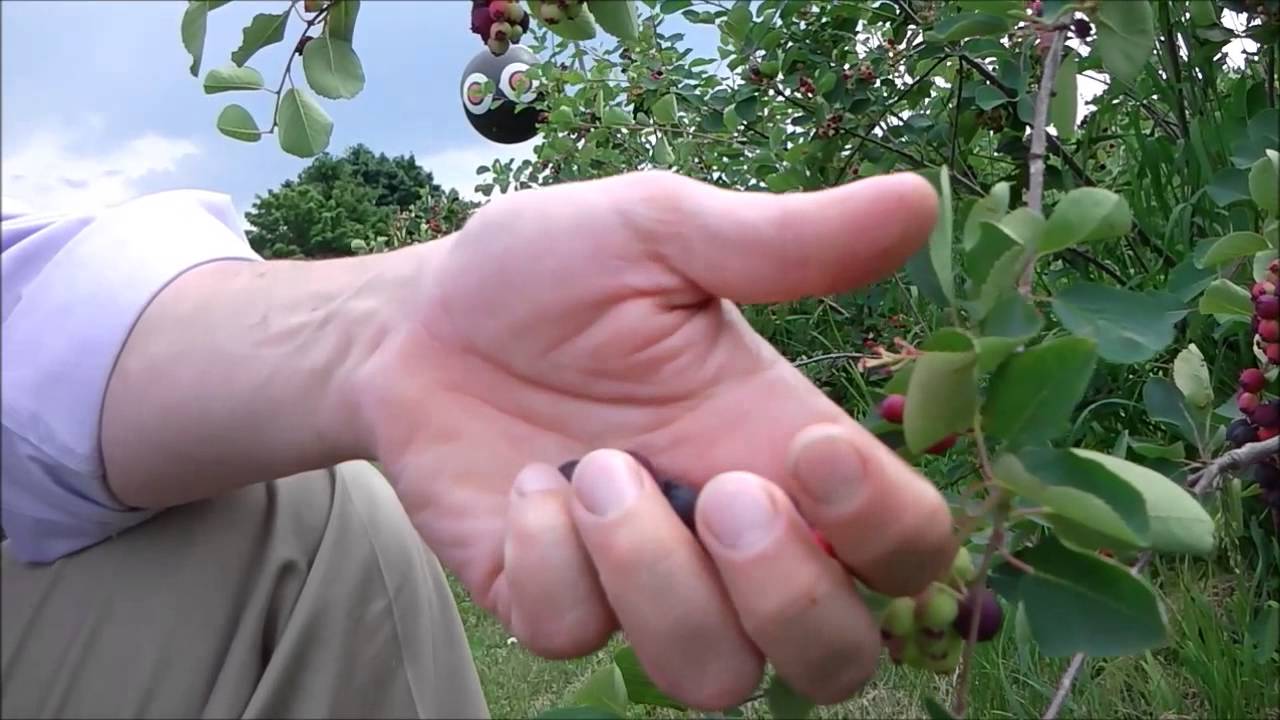In this detailed photograph, a close-up shot captures a man’s left hand resting on his knee, with his fingers curled and holding several blueberries while reaching towards a plant with green leaves and reddish-blue berries. The man is wearing beige pants and a white shirt with the sleeves rolled up. His forearm rests comfortably on his knee. The background reveals a countryside scene with abundant foliage, including bushes bearing dark red and green berries. In the top left corner of the image, a blue sky with scattered clouds is visible. Intriguingly, there is a round black object resembling a balloon or perhaps a spherical camera with yellow and white circles positioned towards the middle-left, adding an element of curiosity to the scene.